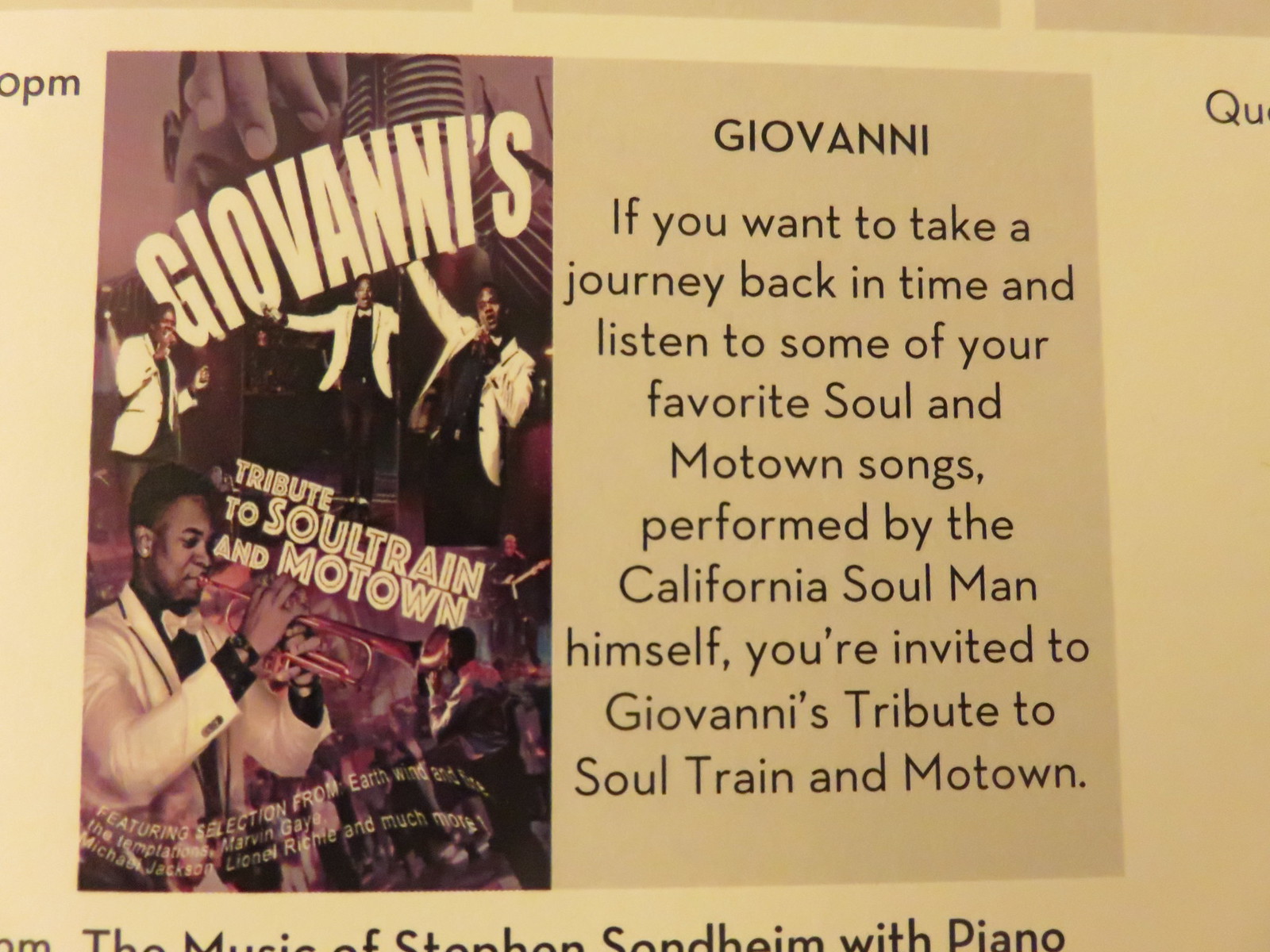The image is a vibrant poster advertising a musical event titled "Giovanni's Tribute to Soul Train and Motown." Dominating the left side of the poster is a purplish collage featuring a black man in a white suit or bow tie, captured in various dynamic moments playing the trumpet and singing into a microphone. Above this collage, large yellow text announces "Giovanni's," followed by smaller yellow text that reads "tribute to Soul Train and Motown." On the right side, set against a gray background, there is black text stating: "Giovanni. If you want to take a journey back in time and listen to some of your favorite Soul and Motown songs performed by the California Soul Man himself, you're invited to Giovanni's Tribute to Soul Train and Motown." Below this, partially visible, is another piece of text, hinting at an additional program related to the music of Stephen Sondheim with piano. The entire background of the image is a lively shade of yellow, adding to the overall appeal and energy of the poster.